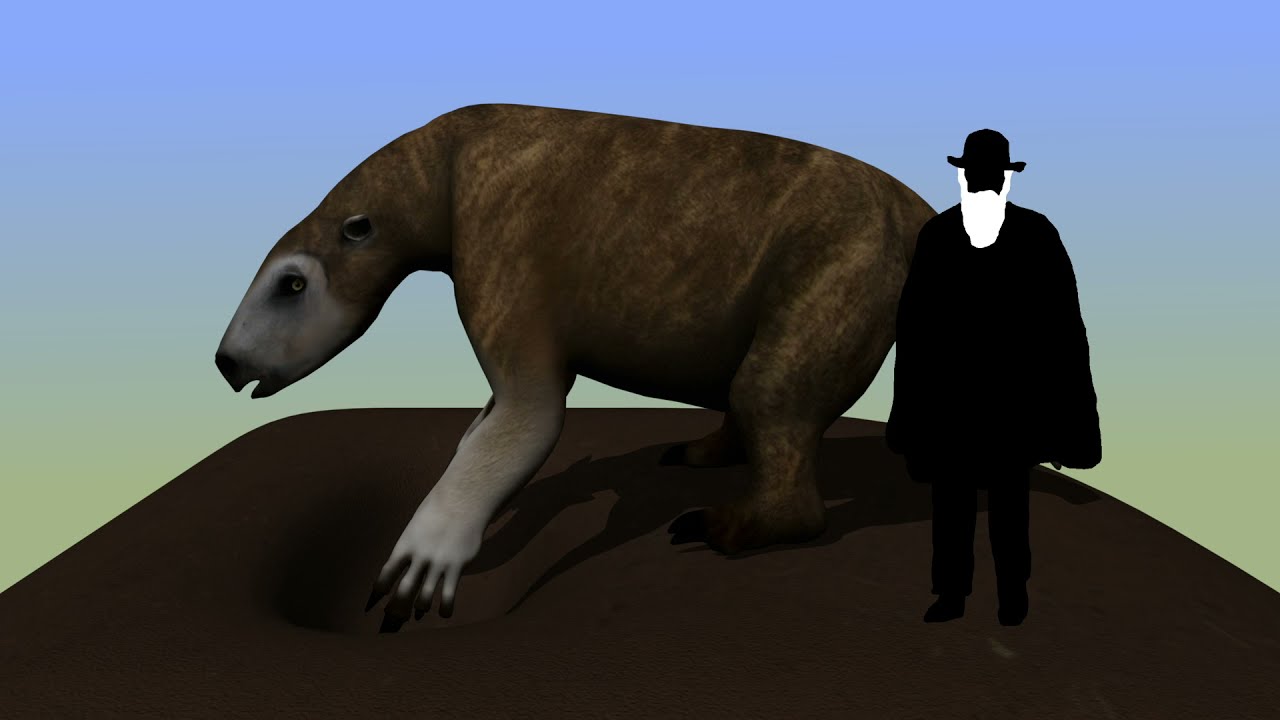The image depicts a low-quality, 3D-generated representation of a massive, mythical or prehistoric creature resembling a giant sloth. This colossal animal, facing left and standing on four massive limbs, has a brown body with light brown streaks, a grey head, and grey front paws. Its elongated snout features a black, almost beak-like mouth, while small brown ear holes are situated behind its eyes. The creature appears to be on a large, brown, rock-like formation with minimal texture. Above, the sky transitions from blue to green. To the right, a black silhouette of a man, possibly representing Charles Darwin, stands. This figure, bearing a white beard and wearing a black hat and shawl, serves to illustrate the creature's enormous size. Notably, the silhouette lacks eyes and the full structure of the creature's tail is obscured from view. The sloth's front limbs have four visible digits and possibly a fifth claw-like thumb that is hidden.